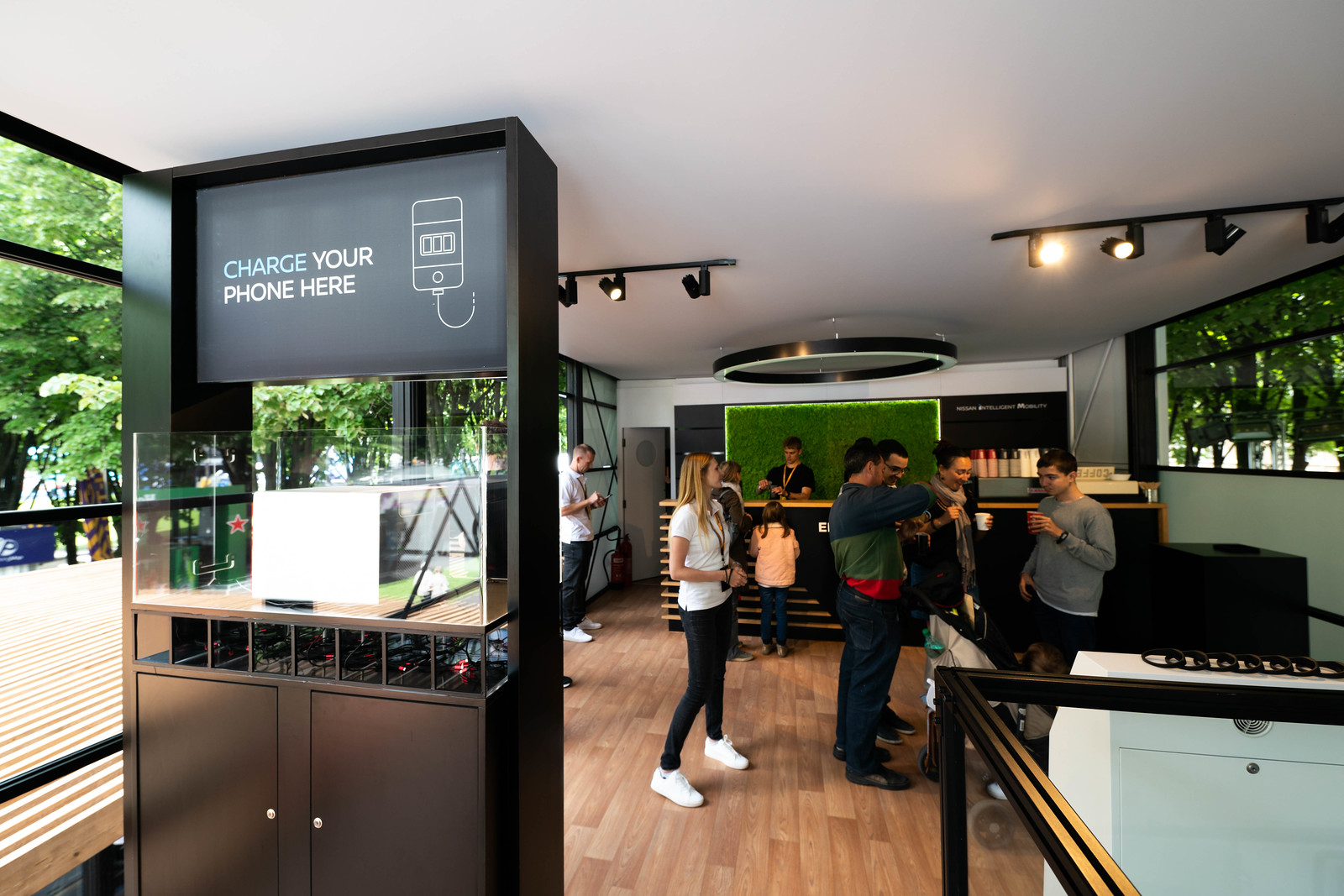In a modern indoor cafe with a light brown wooden-paneled floor, large windows stretch along the left side, filling the space with natural light. At the left foreground, a sleek black cabinet displays the text "charge your phone here," with an outline of a phone and charger on its right side and multiple charging stations below, some with red indicator lights. 

The center of the image is filled with a group of men and women holding cups of coffee, socializing near a child and a parent who stand close to the serving area. This serving area, a desk counter, is manned by a barista wearing a black t-shirt complemented by a black and red lanyard. Above the barista, a circular light fixture illuminates the workspace, while studio-like lights hang from the ceiling. 

The back corner of the room features a fake grass wall adorned with lights, enhancing the modern aesthetic. The barista appears to be preparing coffee amidst neatly arranged plastic cups that line the back corner, underscoring the cafe's attention to detail.